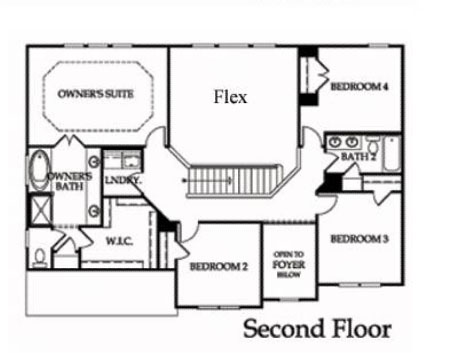Detailed Caption: 

The image is a detailed floor plan of the second floor of a house, depicted in black and gray writing. Predominantly rendered in black, the gray highlights the entry points, likely representing the doors and front part of the house. The floor plan prominently shows an expansive "Owner's Suite" situated towards the left side. This suite encompasses a spacious sleeping area, a generous owner's bath, and a large walk-in closet. The owner's bath includes a separate toilet area and is adjoined by a conveniently placed laundry room.

Centrally located on the floor plan is a "Flex Area," which serves as a transitional space connecting the owner's suite to the other bedrooms. Directly across from the owner’s suite lies "Bedroom 4," which shares a Jack-and-Jill bathroom with "Bedroom 3." This shared bathroom features dual sinks, a spacious bathtub, and a toilet.

In addition to these bedrooms, "Bedroom 2" is situated near the walk-in closet of the owner's suite. The design also incorporates an open-to-below area, creating a balcony effect that provides a view of the foyer on the first floor. An arrow on the floor plan indicates a staircase leading down to the first floor. This detailed layout offers a comprehensive view of the second floor's functional and spacious design.